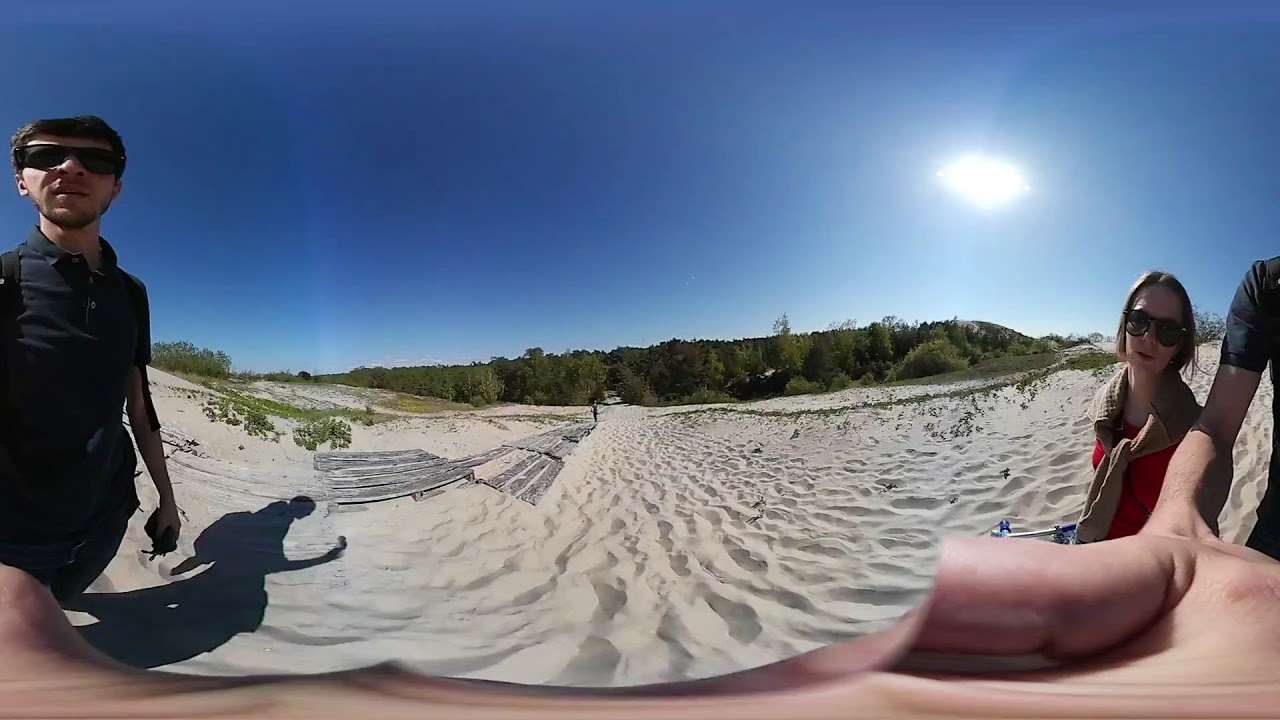This horizontal rectangular image, distorted by an unusual wide-angle or 360-degree lens, captures a beach scene with two people standing side by side. The man on the left, sporting dark sunglasses, a black short-sleeve polo shirt, and shorts, has short dark hair and facial hair. His outstretched arm and hand, holding the camera, dominate the lower portion of the image, creating significant distortion. The woman on the right, also wearing sunglasses, has a sweater tied around her shoulders. The sandy landscape extends back to a horizon lined with sparse vegetation and trees. The sky overhead is a deep blue, indicating daylight, with the sun positioned off-frame to the right, casting shadows on the sand. Alongside the sand, the image suggests the presence of some wooden elements, possibly remains of stairs or a platform, blending into the beach setting.